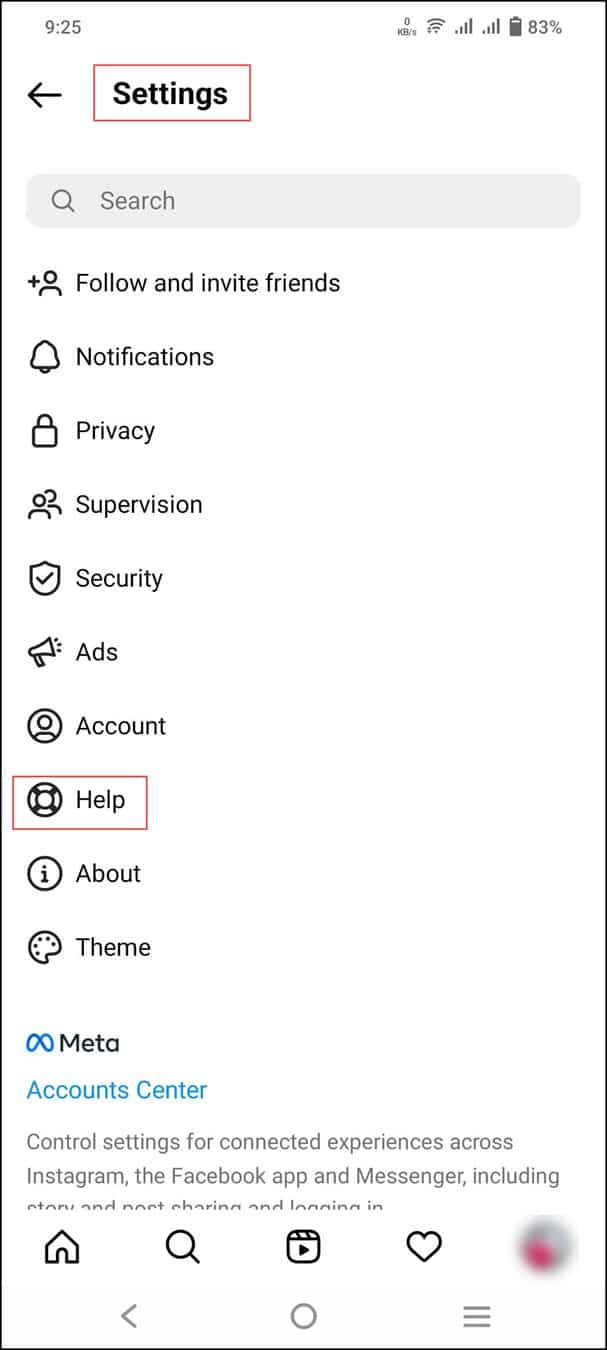This digital image displays a settings interface for a social media application. The top of the screen shows the current time, "9:25," and a battery icon indicating 83% charge. Adjacent to these icons is a search button for navigation.

The primary settings options are listed below, starting with "Follow and Invite Friends," followed by "Notifications," which features a notification bell icon. The "Privacy" and "Supervision" settings come next, with the "Security" section marked by an image of a shield with a black checkmark.

Further down, the "Ads" and "Account" settings are visible, followed by a prominently outlined red rectangle containing a "Help" button, which is illustrated with a life jacket icon. The "About" button and "Theme" button are located below these options.

At the bottom of the screen, the "Meta" logo is displayed alongside an "Account Center" section. This section provides options to control settings for connected experiences across Instagram, including links to the Facebook app, Messenger, and a website. Additional options are available for managing messaging, story and post sharing, and login settings.